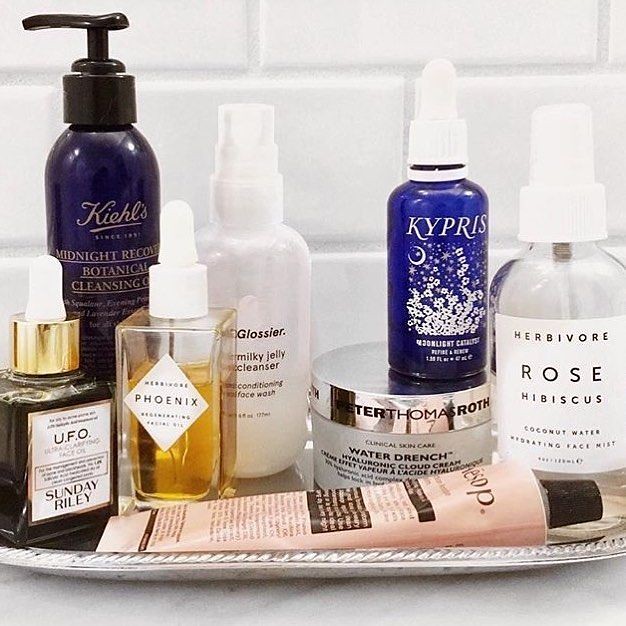This photograph, slightly taller than it is wide, showcases a meticulously arranged collection of beauty products against a backdrop of Subway-style white tiles. The products rest on a marbled countertop, adding to the sophisticated aesthetic.

Central to the image is a polished silver tray holding seven distinct beauty product containers from various brands. Among these, a midnight blue bottle of Kiehl's Midnight Recovery Botanical Cleansing Oil stands out with its black dispenser oriented left. Adjacent to it is Sunday Riley's UFO Ultra-Clarifying Face Oil, along with Phoenix, another product by the same brand.

Also featured are items from Kypris and Herbivore, specifically the Rose Hibiscus Hydrating Face Mist. There's a jar of Water Drench Hyaluronic Cloud Cream, notable for its hydrating properties. A uniquely colored coral pink tube of cream lies on its side, adding a pop of color to the arrangement.

The deliberate positioning of these products suggests an artful display, emphasizing their aesthetic appeal rather than functional placement inside a medicine cabinet.